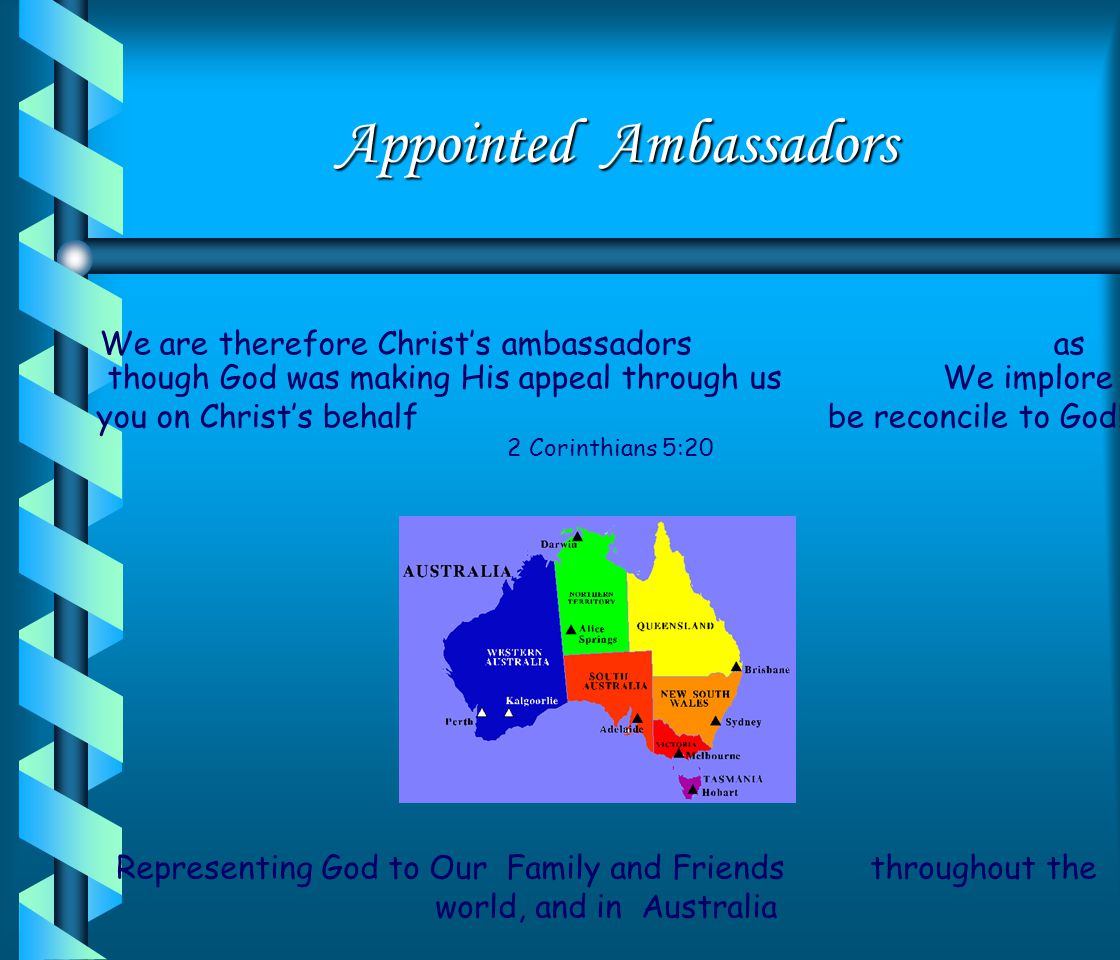The image appears to be a PowerPoint slide featuring a gradient background that transitions from dark blue at the bottom to normal blue at the top. Along the left edge is a dark blue vertical pole with a light blue, digitally-styled ribbon spiraling around it, resembling the spine of a spiral-bound notebook. At the top of the slide, the title "Appointed Ambassadors" is prominently displayed in white text.

Below the title, there is a section with several Bible verses rendered in dark blue text. The key verse highlighted is, "We are therefore Christ's ambassadors, as though God were making his appeal through us. We implore you on Christ's behalf: Be reconciled to God" (2 Corinthians 5:20). Additionally, there are some text elements that are truncated and not fully legible.

Centrally positioned is a detailed map of Australia, divided by regions such as Queensland, New South Wales, and Western Australia, each distinguished by vibrant colors like blue, lime green, yellow, and red. Underneath the map, in dark blue text, it reads, "Representing God to our family and friends, world, and in Australia." On the right side of the slide, there is partial text that begins with "throughout the," but it is cut off and incomplete.